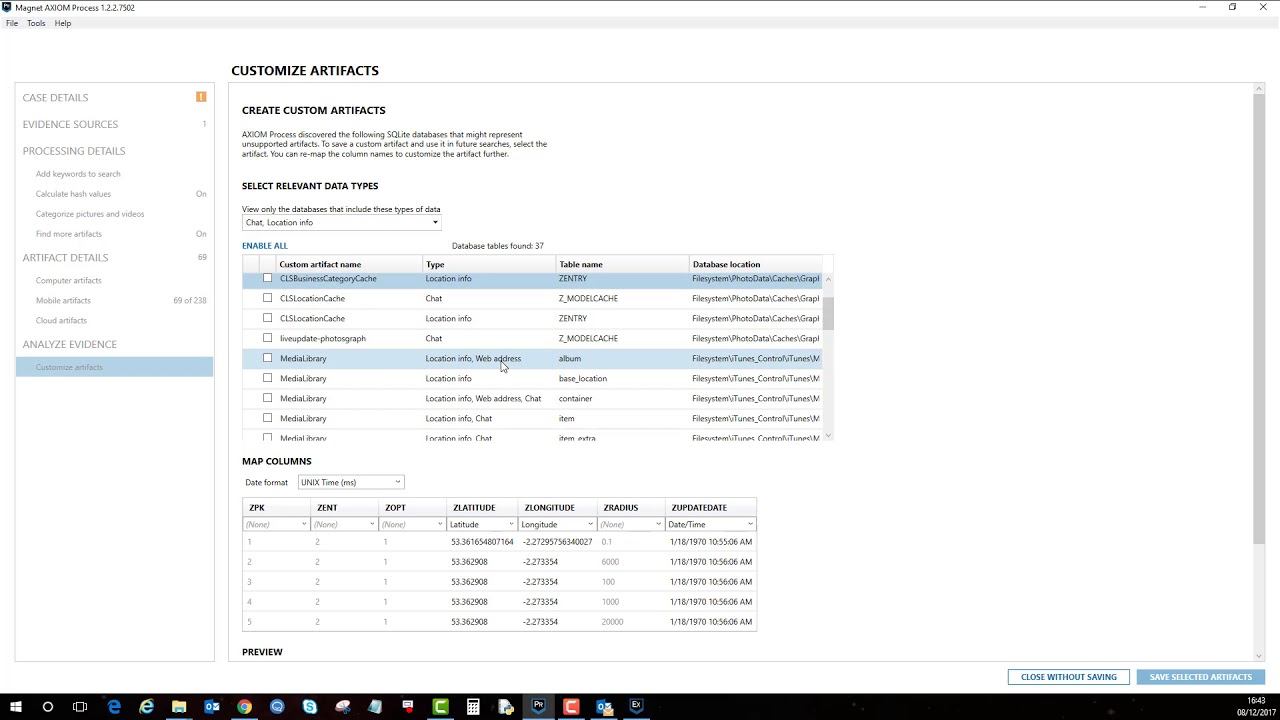The image captures a detailed screen from a website interface. At the top, there is a thin white bar with small black font that includes options such as "File," "Tools," and "Help," alongside window control icons: a minus sign, a window sign, and an 'X' for closing the window. 

Below, a vertical white side menu features an orange icon followed by gray text headings: "Case Details," "Evidence Sources," "Processing Details," each with indiscernible sub-bullet points. Further down are "Artifact Details" and "Analyze Evidence."

In the main section at the top, bold black headers read "Customized Artifacts" and "Create Custom Artifacts," supported by a paragraph of black text. Below, it says "Select Relevant Data Types" accompanied by a white drop-down menu. A list follows with black text items next to white checkboxes, arranged into four columns.

Underneath, there's another section labeled "Map Columns," featuring a drop-down menu, followed by a chart with black text and additional pull-down menus. At the bottom, options "Preview" and blue buttons for "Close Without Saving" and "Save Selected Artifacts" are present.

The bottom of the image includes a black toolbar hosting several icons: Internet Explorer in blue, a manila folder, Chrome, a calculator, other blue and green icons, a red icon, and the Windows white flag which also displays the date and time.